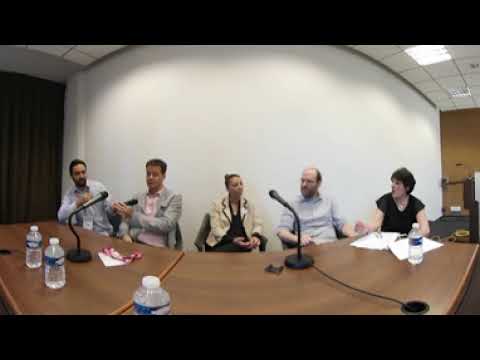The image captures a business meeting in a well-lit conference room with white walls and white ceiling tiles fitted with fluorescent lights. The central focus is on a wide, curved wooden table arranged in a half U-shape. There are five people — two women and three men — seated along one side of the table, facing the camera. On the far left, a black curtain is visible, while behind the participants, a blank white wall forms the background. 

The participants, dressed in business or business casual attire, are arranged as follows from left to right: a man in a blue shirt, a woman in a tan blazer, a man in a gray blazer, another man in a blue shirt, and a woman in a black shirt. The table features four plastic water bottles, various papers, and two microphones. The woman on the far right, clad in the black shirt, has her hands raised and appears to be the one speaking, while the others listen attentively. Additionally, there is a hole in the wooden table for microphone cords, enhancing the functionality of the setup for the meeting.